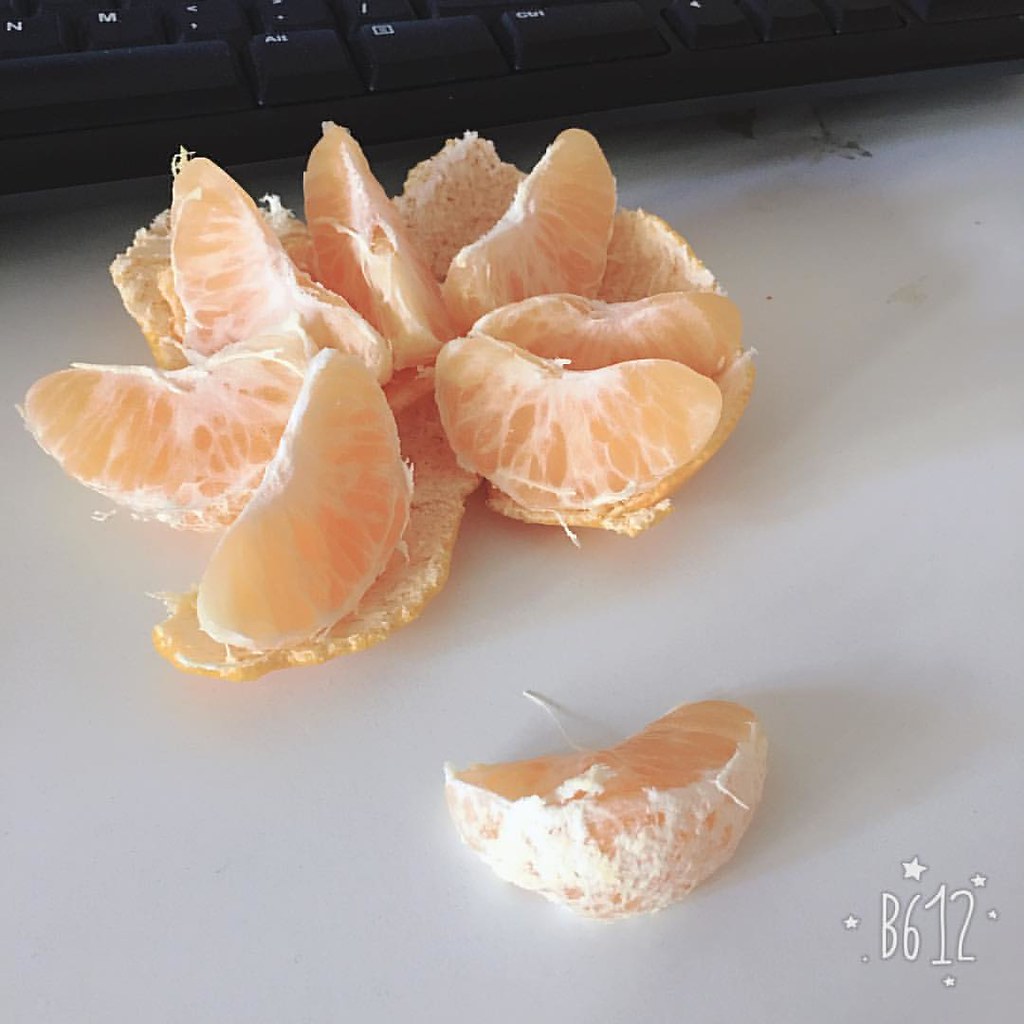An angled close-up image features a peeled orange displayed on a white table, with segments thoughtfully arranged on the intact peel, which is slightly torn on the middle right side. One segment lies independently on its side in the foreground, facing outward. The setting includes a partially visible black keyboard at the top of the frame, showing the N, M, spacebar, and alt keys. At the bottom right corner, the text "B612" appears in white font, surrounded by small stars. The orange segments, still encased in thin membranes and partially covered with skin, are organized in a circular pattern atop the neat, spread-out peel, suggesting a meticulous peel removal.